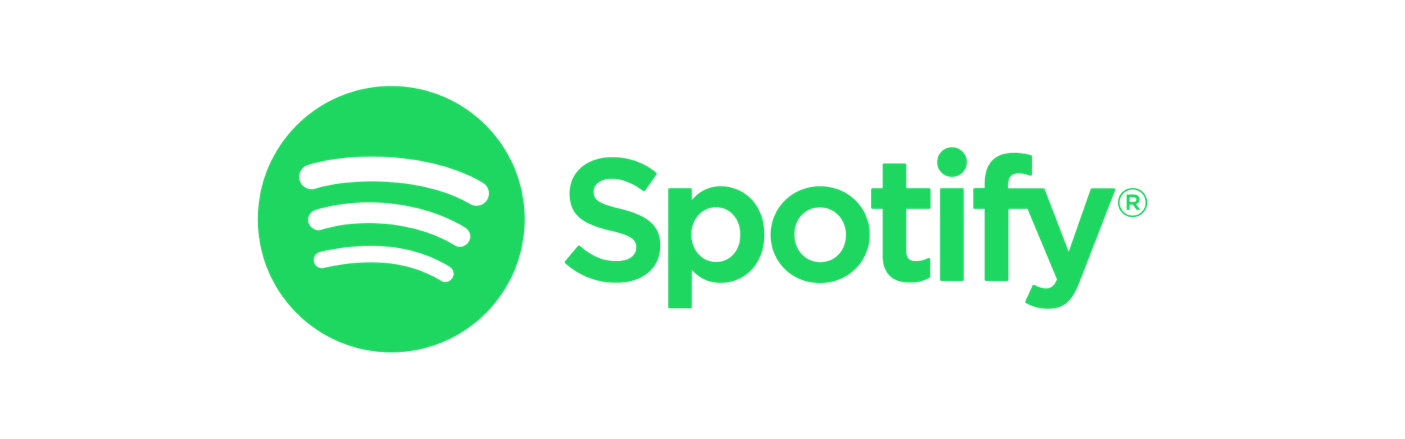This image features the Spotify logo prominently displayed against a plain white background. On the left, there is a green circle containing three white, curved lines that resemble sound waves. These lines are of varying lengths, arranged with the shortest on top and the longest at the bottom. This emblematic symbol is paired with the word "Spotify," written in the same characteristic green as the logo. The text is in a clean, modern font with a capital 'S' followed by lowercase letters, and is positioned to the right of the logo circle. Adjacent to the word "Spotify" is a small registered trademark symbol (®), also in green, further authenticating the branding. Overall, this image closely echoes the official Spotify icon and typeface, making it look suitable for use in advertising or promotional materials.